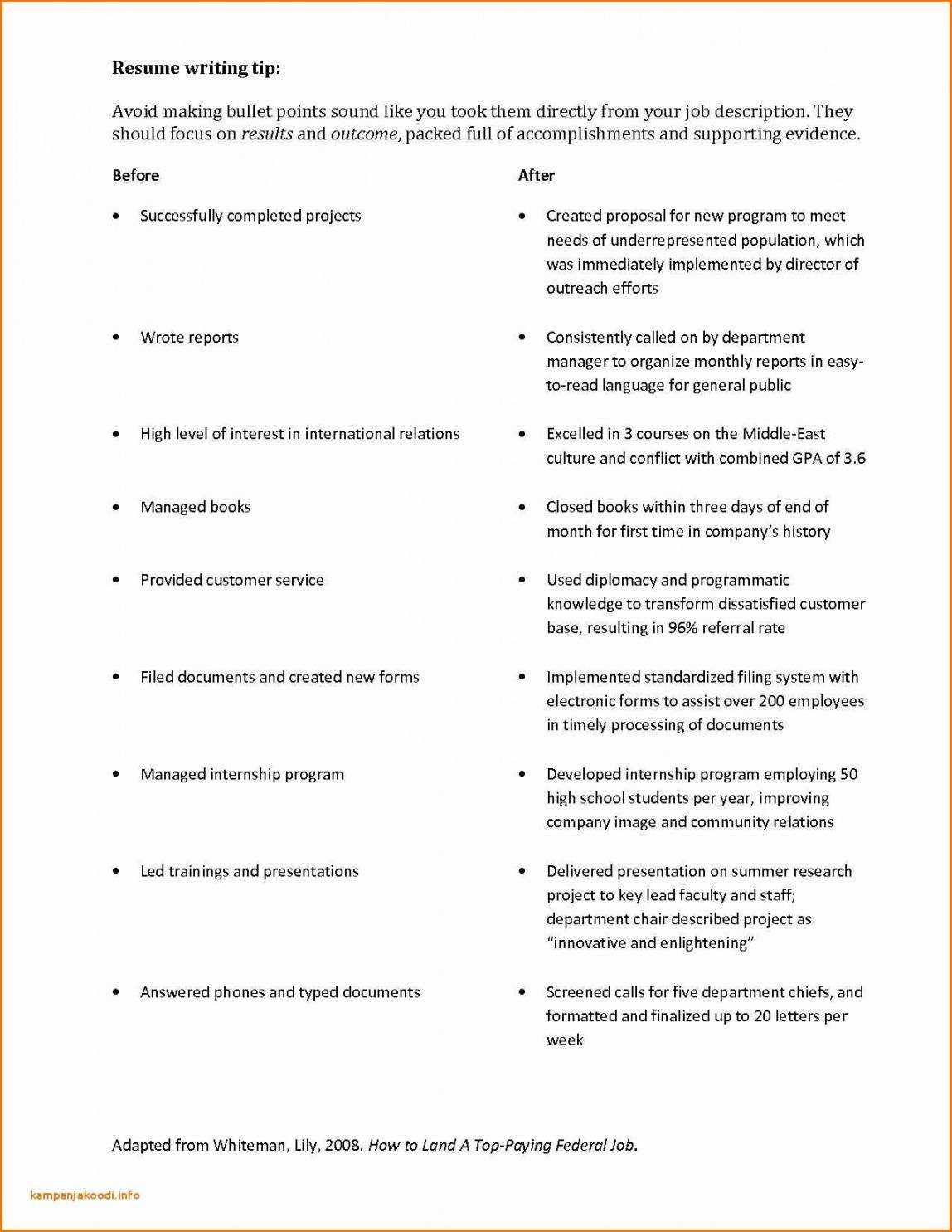**Descriptive Caption:**

This desktop screenshot showcases a professional resume writing tip from a website displayed against a clean, white background. The webpage is bordered by a striking goldish-red line, adding a touch of elegance to the presentation. The central focus of the page is an extensive amount of text, formatted to provide insightful advice on enhancing resume bullet points by emphasizing results and achievements rather than mere job descriptions. The content is adapted from Whiteman Lilly's 2008 guide, "How to Land a Top Paying Federal Job," and is accessible via the URL kampanjakoodi.info.

The visual divides information into two distinct, bulleted columns labeled "Before" and "After." The "Before" column lists common resume entries, such as "Successfully completed projects" and "Wrote reports," while the "After" column transforms these entries into more compelling accomplishments:

- "Created proposal for new program to meet needs of underrepresented population, which was immediately implemented by the Director of Outreach Efforts."
- "Consistently called on department manager to organize monthly reports in easy to read language for general public."
- "Excelled in three courses on Middle East culture and conflict with a combined GPA of 3.6."
- "Closed books within three days of end of month for first time in company's history."
- "Used diplomacy and programmatic knowledge to transform dissatisfied customer base, resulting in 96% referral rate."
- "Implemented standardized filing system with electronic forms to assist over 200 employees in timely processing of documents."
- "Developed internship program employing 50 high school students per year, improving company image and community relations."
- "Delivered presentation on summer research project to key lead faculty and staff; Department Chair described project as innovative and enlightening."
- "Screened calls for five department chiefs and formatted and finalized up to 20 letters per week."

These revised entries showcase tangible evidence of the candidate's impact and contributions in their roles. The screenshot provides a comprehensive comparison, guiding viewers on how to effectively enhance their resumes with a results-focused approach.